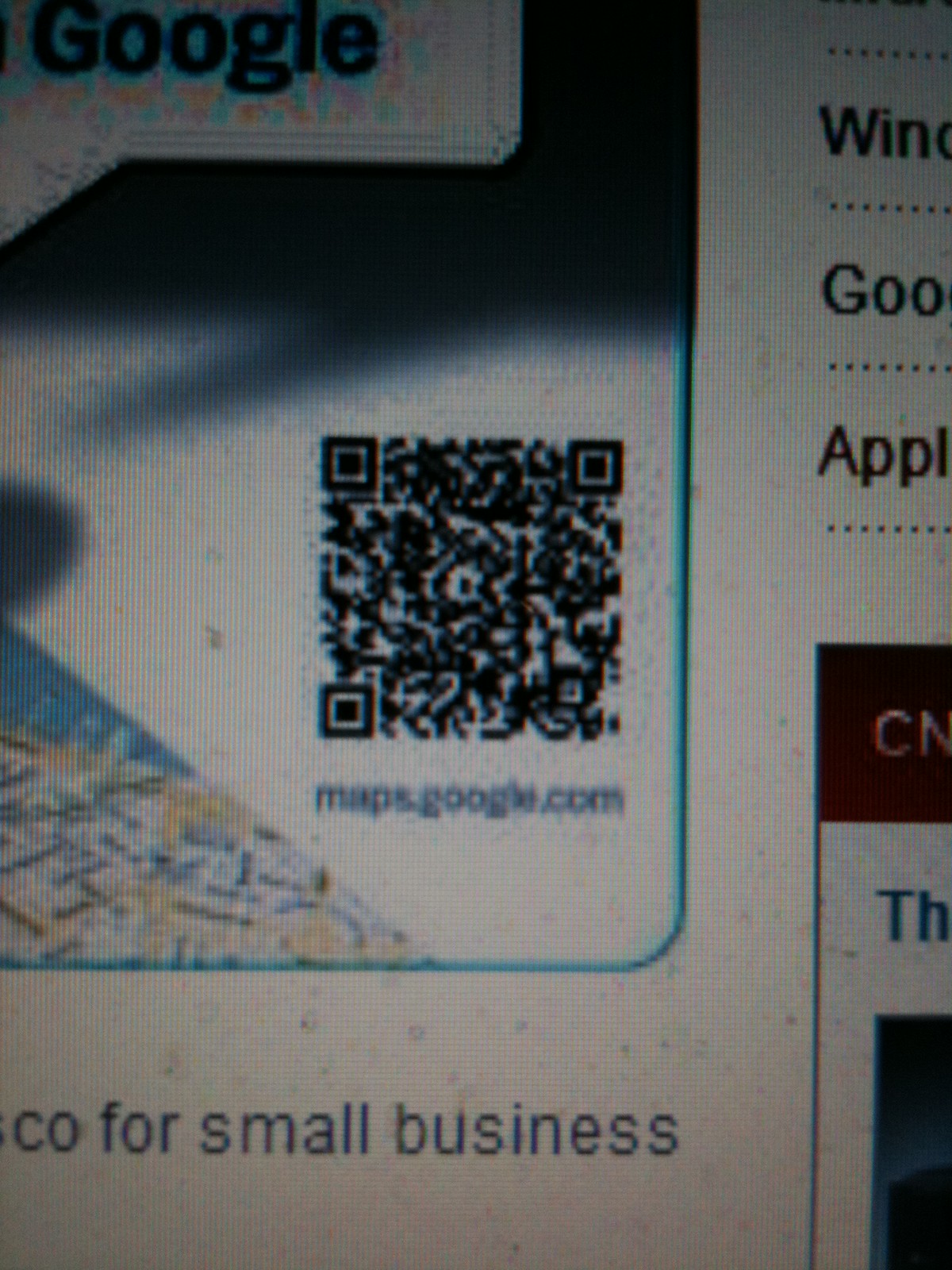This photograph captures a computer screen displaying an image that appears to be around 10 to 15 years old. Dominating the screen is a blue box, with "Google" prominently displayed in a white box at the top left corner. Below this, the screen features a black QR code, likely the focal point of the image. Beneath the QR code, the URL "maps.google.com" is visible. Further down, part of a phrase ending in "CO for small business" can be partially seen, though much of the text is cut off. To the right of the main display, some additional writing is partially visible, accompanied by a small, indistinct red image, hinting at more contextual information. The overall impression is that the photo was taken to capture the QR code for further use or reference.